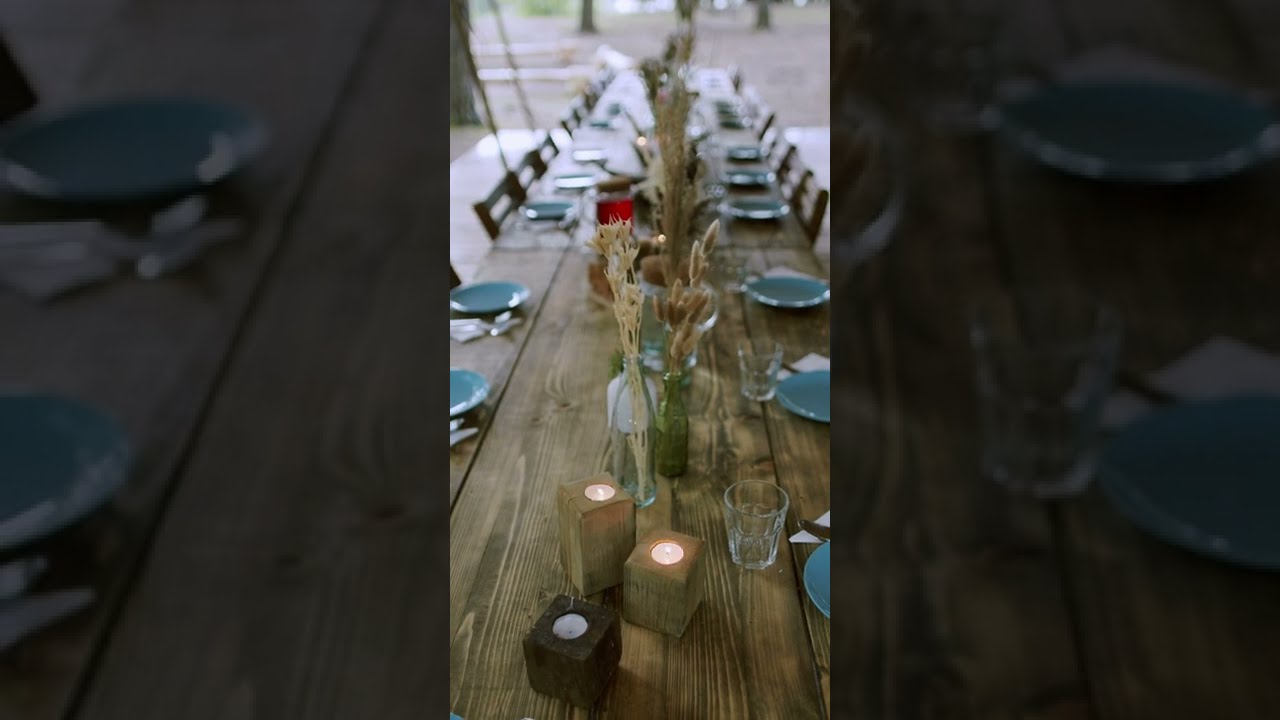In the image, three sections are shown, with the left and right sections being dark zoom-ins of the middle section. The central section reveals a long, rustic banquet table crafted from wooden planks, set up on what appears to be a light gray patio floor, reflecting light in the upper right corner. The table is adorned with green plates, silverware, and short clear glasses placed at each setting, with chairs lined up on both sides. At the foot of the table, there are three square candles; two are lighter brown and lit, while the unlit one, which is the shortest, is a dark brown color. Running down the center of the table are slender flower vases and bottles containing cattails and other ornamental grasses. The background, though blurry, shows a brown dirt area, suggesting an outdoor setting.